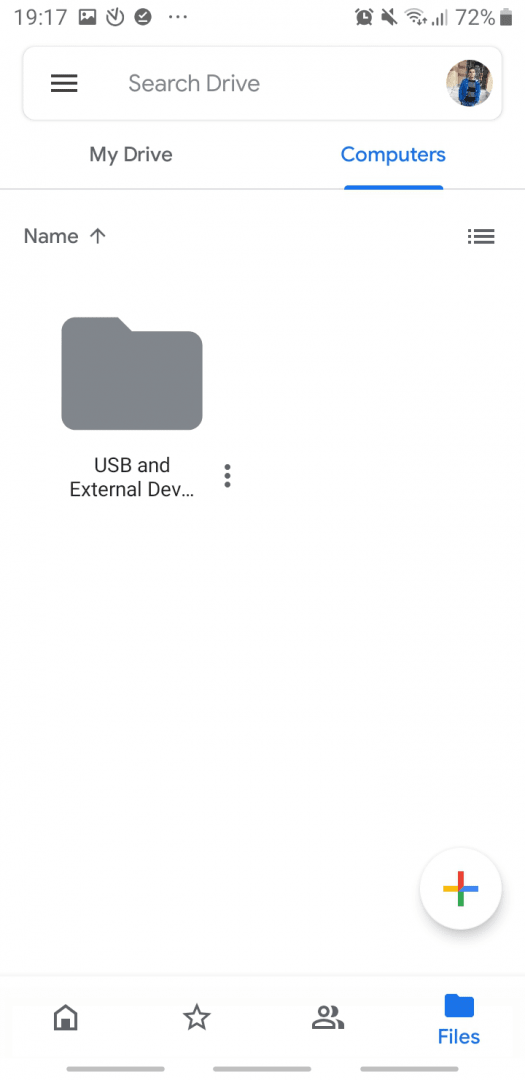A detailed screenshot taken on a mobile device showcases a predominantly white screen with some gray text and various graphic elements. The current time is displayed twice, indicating 9:17 and 19:17. At the top of the screen, there's a thumbnail image of a photo, a checkmark graphic within a circle, and three vertical dots indicating a menu. An alarm graphic is also visible, and notifications have been silenced, as indicated by a notification symbol with an X through it. The screenshot shows that Wi-Fi is enabled with three bars for signal strength, the carrier service is active, and the battery life is at 72%.

In the top right corner, there is a small circular photo of the device owner, a man with dark hair wearing a blue zip-up shirt. Below his photo, there is a search bar, denoted by three horizontal lines. The screen displays the heading "My Drive" in gray text, with "Computers" highlighted in blue. Additional items listed include "Name" with an upward-pointing arrow, "USB and External Devices" with a gray folder icon, and a plus sign denoting Google Plus services.

Icons at the bottom of the screen represent various navigation options: a home graphic, a favorites graphic, and a files graphic highlighted in blue. This screenshot captures a comprehensive view of the user's current mobile interface, showcasing both functional and navigation elements.